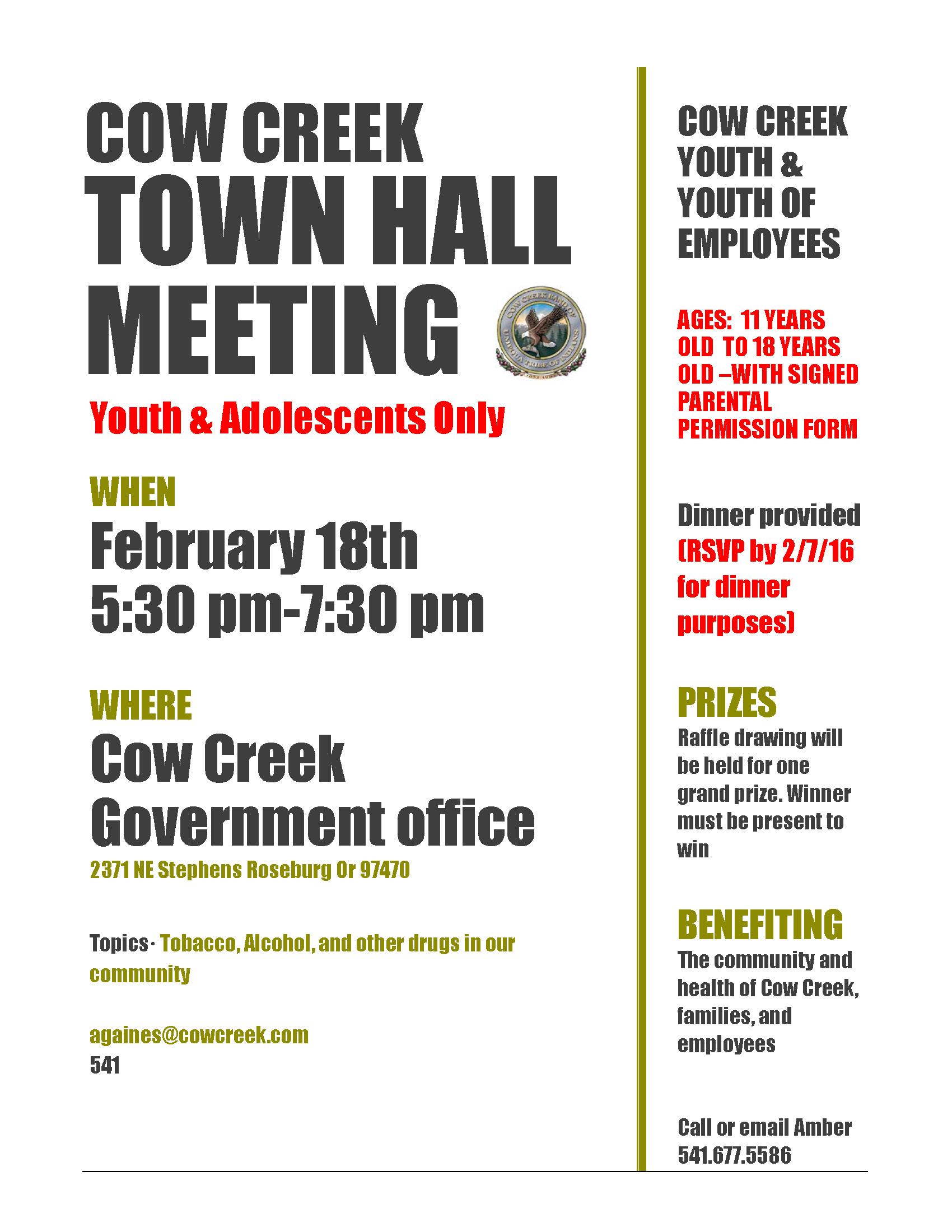**Cow Creek Town Hall Meeting for Youth and Adolescents**

**Date and Time:** February 18th, from 5:30 p.m. to 7:30 p.m.

**Location:** Cow Creek Government Office, 2371 NE Stephens Street, Roseburg, Oregon, 97470

**Audience:** Youth and adolescents, ages 11 to 18 years old, including children of Cow Creek employees. Attendees must have signed parental permission.

**Topics:** Tobacco, alcohol, and other drugs in our community

**Special Notes:**
- Dinner will be provided.
- Prizes will be awarded, including a raffle drawing for one grand prize. The winner must be present to claim their prize.
- RSVPs are required by February 7th, 2016 for dinner purposes.

**Contact Information:**
- For RSVPs and inquiries, contact Amber at 541-677-5586 or via email at againes@cowcreek.com.

**Purpose:** To benefit the community and enhance the health of Cow Creek families and employees.